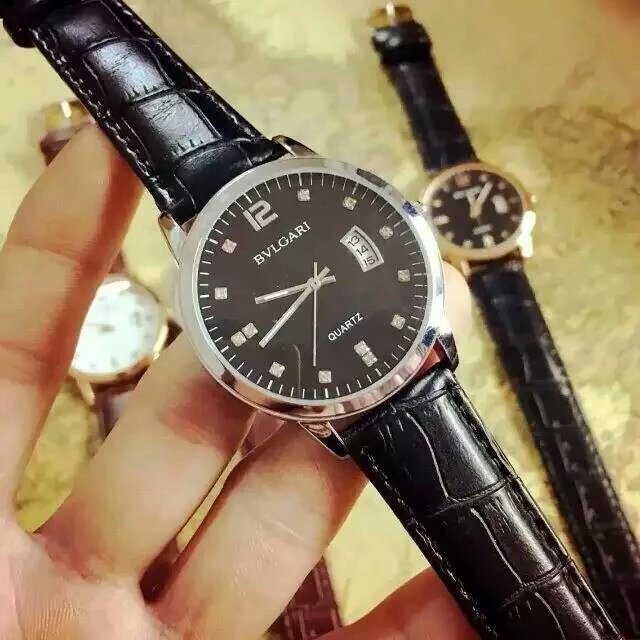This image captures a detailed view of a Bulgari wristwatch being held by a person's left hand, with their palm and the underside of their fingers supporting the watch from the bottom left corner. The watch, which features a black, alligator-style pressed leather band with visible stitching and horizontal lines, has a circular face encased in a shiny silver metal housing. The watch face is black with the brand name "BVLGARI" prominently displayed below the number 12.

The watch's dial displays the time as approximately 9:43, with the second hand just past the seven, indicating around 36 seconds. The number 12 is the only numeral on the face, with the remaining hours marked by inlaid diamonds; the 6 and 9 positions are distinguished by two diamonds each, arranged radially and vertically, respectively. Below "BVLGARI," the word "quartz" is visible, along with an open-faced dial showing the date, which highlights the 14th but also shows the 13th and 15th.

In the blurry background, there are additional watches on what appears to be a granite counter. Among them, a few have brown bands, and one has a black band, adding to the watch collection's variety but remaining indistinct due to the image's depth of field.